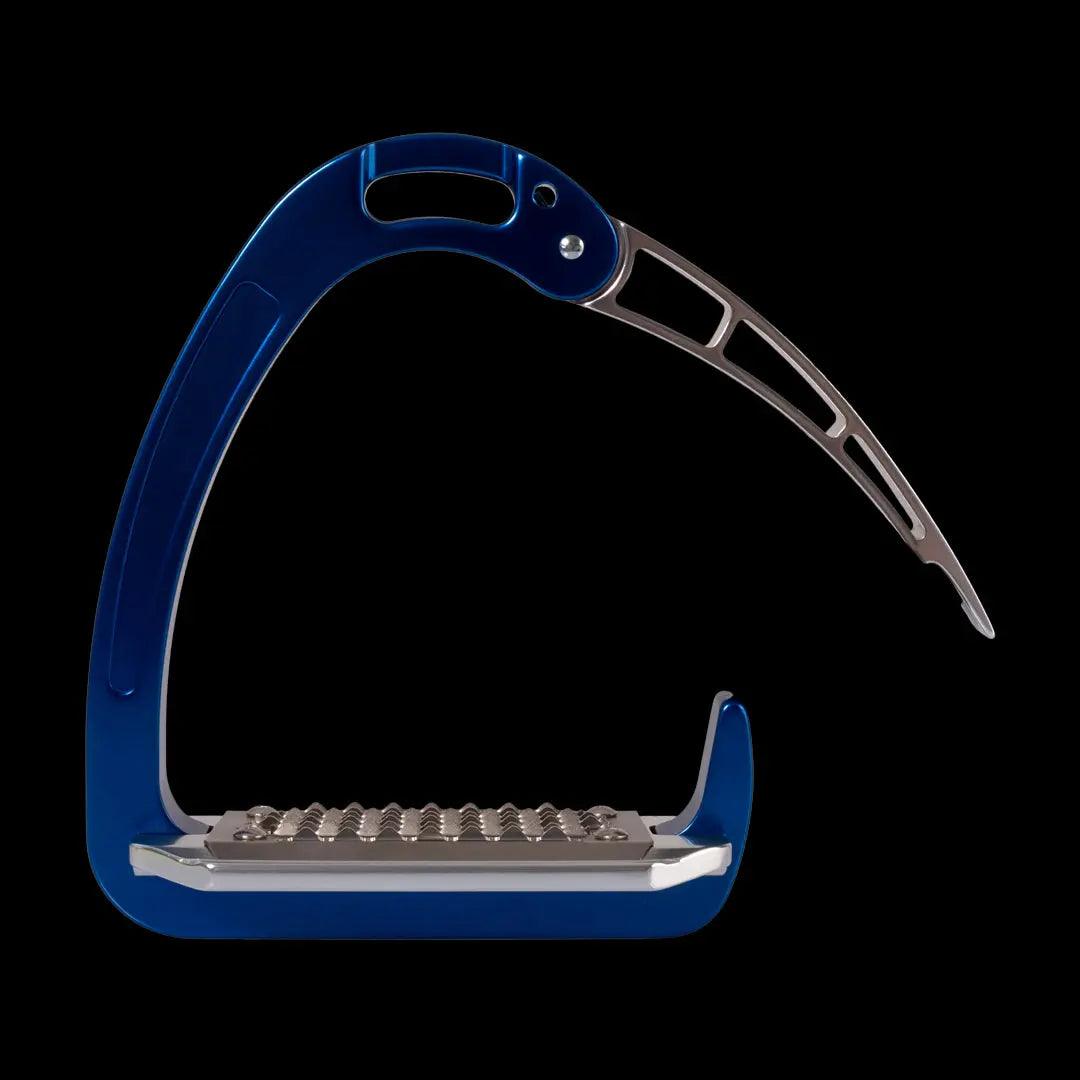This image depicts a blue and chrome metallic device, meticulously placed against a black background that gives it an almost ethereal, floating quality. The device, resembling a cross between a tool and a sculptural piece, features a curving structure reminiscent of a large carabiner. Its architecture is predominantly a medium blue hue, with sections of silver chrome that exhibit a textured, bumpy pattern. The device takes on a C-shape, with the top part curving down into a slightly hooked form, and a flat base that curves upwards towards a bumpy, rectangular plate. This plate appears to serve a stabilizing or gripping function. The chrome blade-like element at the top features a screw, suggesting it can be folded in, enhancing the device's versatile, almost mechanical elegance. The overall aesthetic, with its precise lines and metallic sheen, lends the piece an intriguing sculptural quality that blurs the line between functionality and art.